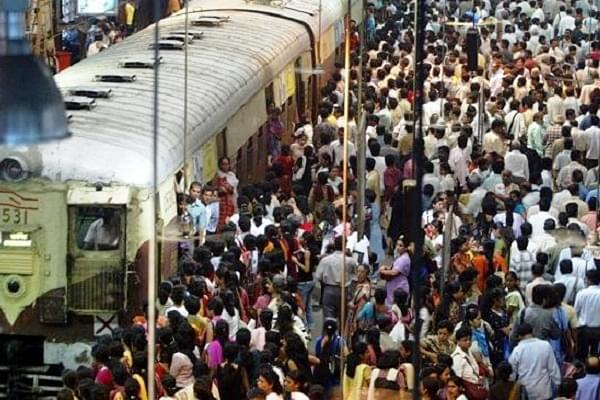The image depicts an exceptionally crowded outdoor train station, likely located in India or Pakistan. The scene is captured from an aerial perspective, showcasing a sea of people densely packed to the right side of the frame, leaving barely any space between them. On the left side of the image, there is a greenish-colored train with a white roof, featuring the number 531 prominently displayed at its end. The train, appearing old and worn out, has passengers hanging out of its doors and windows, suggesting it is already full. The front of the train is at the left bottom of the image, extending towards the top. The bustling crowd, comprised of people in various colored shirts, creates a mosaic of colors against a backdrop that primarily consists of off-yellow, green, white, and black hues. Despite occasional light poles, the overwhelming impression is one of intense congestion, where the platform or sidewalk is barely visible amidst the throng of individuals either waiting to board or having just alighted from the train.